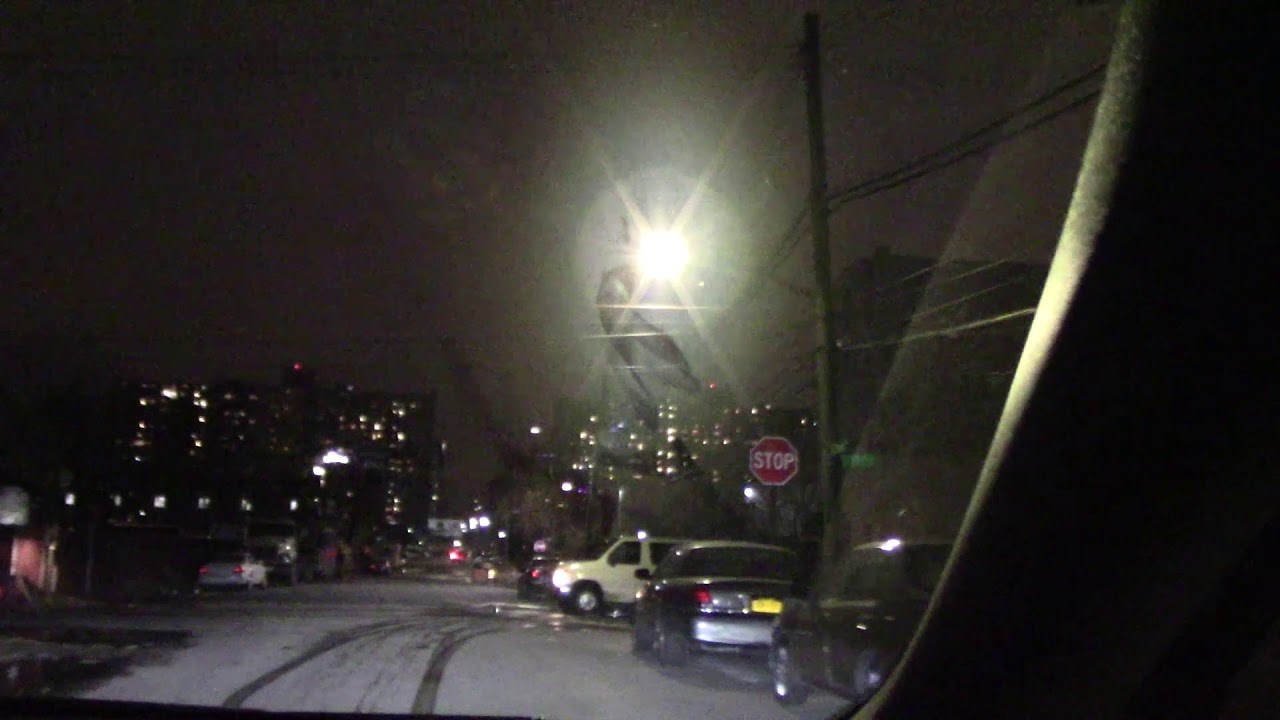This night-time photograph, captured from inside a vehicle, offers a partial glimpse of the car's door frame through the windshield. The background features densely packed, apartment-like buildings with several illuminated windows casting an amber glow. At the top of one building, a red light stands out against the night sky. Parked along one side of the street are several cars, including two darker ones and a white car with its headlights on. In the foreground, a red and white stop sign and a green street sign are clearly visible. On the opposite side, a reddish building can be seen, along with black marks scarring the street's surface. The image also contains subtle lens flare, adding to the night-time ambiance.